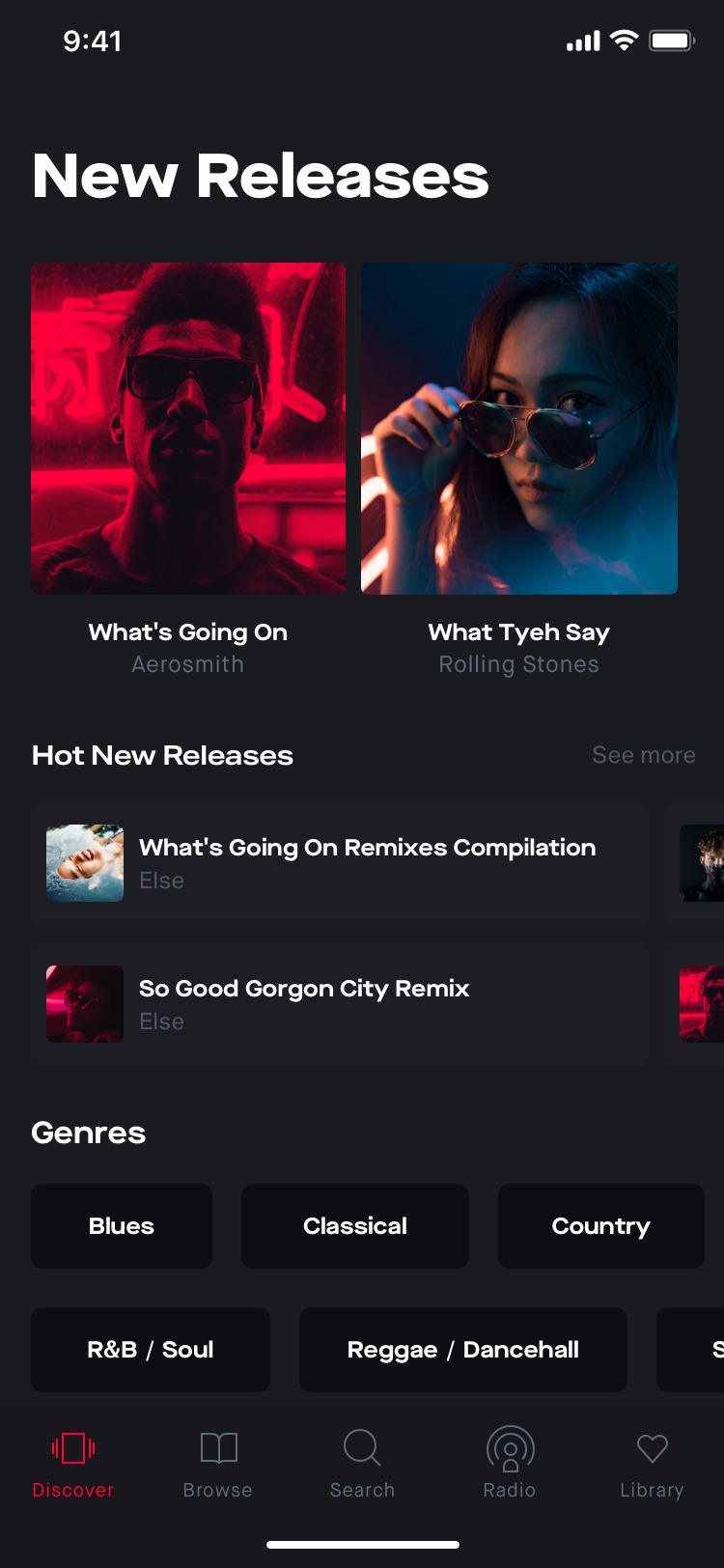The image is a screenshot from a mobile app or website, with an aspect ratio approximately three times as high as it is wide. The entire background is black. At the top left, in large bold white font, it reads "New Releases," with both the 'N' and 'R' capitalized. 

Below this heading are two square images. The one on the left features a red and black color palette, depicting a shadowy figure resembling a Facebook icon. Below this image, it says "What's Going On" and "Aerosmith." To the right, another square shows a young girl pulling down her sunglasses glaring intently at the viewer, with the text "What They Say" and "Rolling Stones" below her.

Further down the screen, on the left, the text "Hot New Releases" appears, followed by a square whose content is difficult to discern, but the text nearby mentions "What's Going On in the Cisco Population" and "ELSP." Another distinct album cover follows, with a black and red color scheme, stating "So Good, Morgan City Remix" and again "ELSP."

At the bottom, there is a section listing genres in white text, with buttons for "Blues," "Classical," "Country," "R&B," "Soul," "Reggae," and "Dancehall."